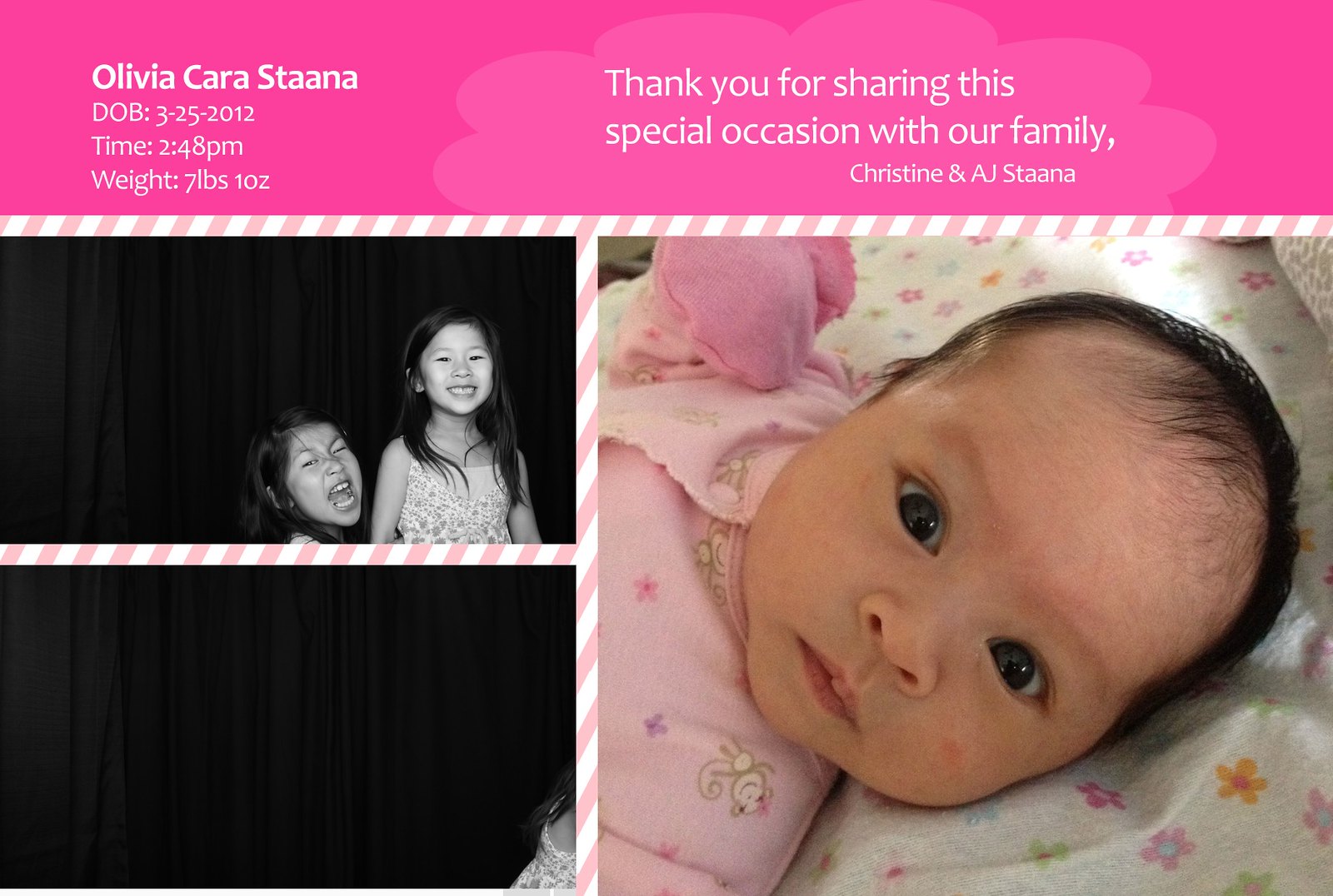This image is a beautifully detailed collage comprising three distinct photos celebrating the birth of Olivia Cara Stana. At the top of the collage is a pastel pink banner adorned with white text. On the left side of the banner, it provides key birth details: "Olivia Cara Stana DOB 3-25-2012 Time 2:48 PM Weight 7 lbs 10 oz." To the right, in the same pink banner, a message reads, "Thank you for sharing this special occasion with our family," followed by "Christine and A.J. Stana" in smaller lettering below.

Beneath this banner and separating the photos is a decorative horizontal strip featuring alternating pastel pink and white stripes. The first section on the left contains two equal-sized black-and-white photos stacked vertically. The top photo shows two young girls with a dark gray background. The girl on the right is smiling, standing tall in a flowered dress, while the girl to her left, with a side-parted hairstyle, is shorter and has her mouth open in a playful expression. The photo below is mostly dark, with a glimpse of the lower girl’s hair, part of her bare back, and her flowered dress visible in the bottom right corner.

Occupying the right half of the collage is a larger, full-color photo of the newborn, Olivia. She has dark hair, a receding hairline, and dark curious eyes, gazing directly into the camera. Olivia is wearing a pink onesie adorned with charming little animal caricatures, pastel flowers, and butterflies. Her right arm is folded, showcasing a pink mitten on her tiny hand. She is laying on a white sheet decorated with multicolored flowers in hues of orange, pink, purple, yellow, and green, adding a lively and cheerful touch to the announcement.